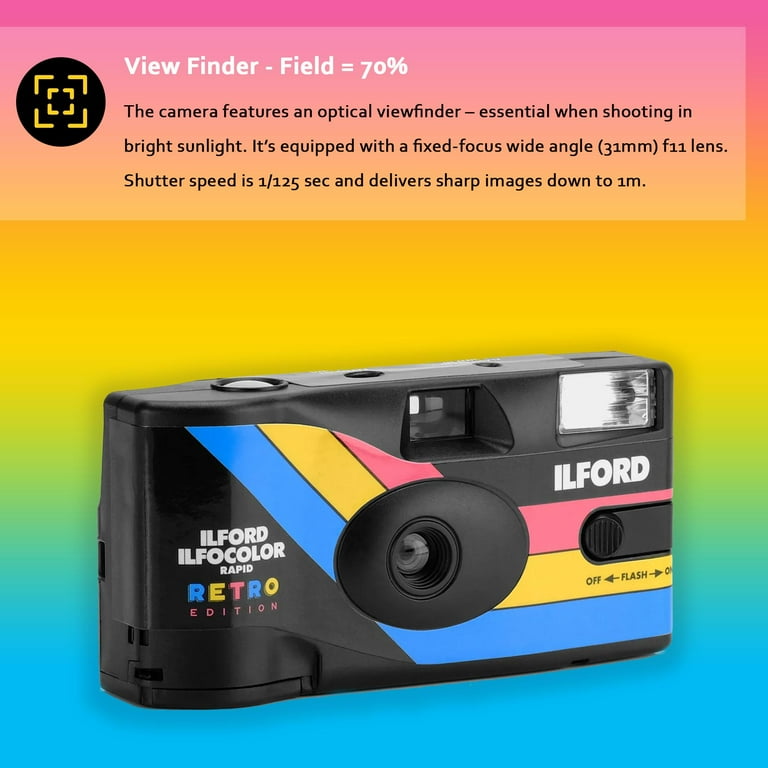The advertisement showcases a retro-style disposable camera centered against a vibrant, gradient rainbow background that transitions from blue at the bottom through green, yellow, orange, red, and finally to purple and pink at the top. The composition is square, with equal length and size for all four sides. At the very top, a semi-transparent white rectangular banner contains text: in white Letters, “Viewfinder minus field equals 70 percent.” Below that, the text in black reads, "The camera features an optical viewfinder, essential when shooting in bright sunlight. It’s equipped with a fixed focus wide-angle 31 millimeter F11 lens, shutter speed is 1.25 sec and delivers sharp images down to 1M." 

The camera itself is mainly black and prominently positioned, facing directly at the viewer. It includes colorful stripes—yellow, blue, and red—along with a silver rectangular area next to the lens, presumably for the flash. The camera is marked with the brand name "Ilford" and is part of the "Ilfo-color-rapid" series. The overall aesthetic of the image nods to the nostalgic appeal of old-fashioned disposable cameras, enhanced by the lively, rainbow-colored backdrop that evokes a sense of playful nostalgia.